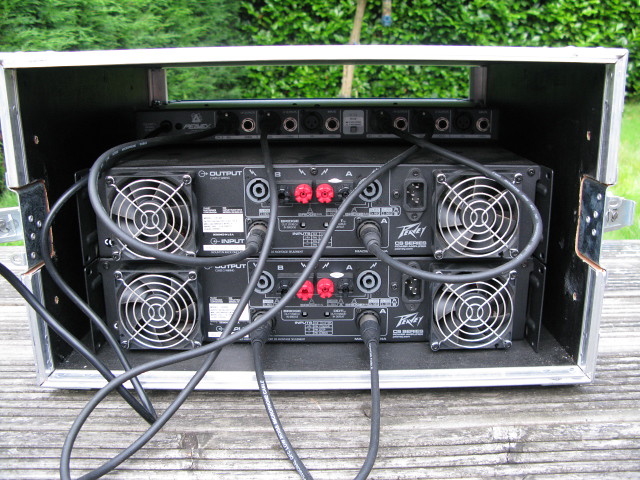This color photograph, taken outside in bright daylight, captures a detailed view of an electrical setup on a light grayish-toned wooden park bench or picnic table. Central to the image is an open, white metal container housing two stacked electronic devices that appear to be sound systems or amplifiers. These devices feature various knobs and buttons in the center, including two prominent red ones. Numerous cables and cords are emerging from the back of these amplifiers, threading through the top section of the metal box.

Each amplifier has a fan on both the left and right sides, distinguishable by their round, concentric circles design. The topmost device displays the term "output" in the upper left, while a label indicating "input" is found below a section filled with text. Another label reads "P-R-P-R-V-E-Y," and the word "penly" is noted on the bottom right device. These labels and components are surrounded by an array of connectors, including red and black knobs and cables, some of which sweep towards the viewer.

The background features a soft focus view of lush, bright green trees and a grassy lawn, contributing to the outdoor setting. The entire scene is framed by the wooden table's light, weathered surface, complete with horizontal black lines. This detailed outdoor photograph emphasizes the intricate wiring and complex design of the electrical equipment against the vibrant, natural backdrop.